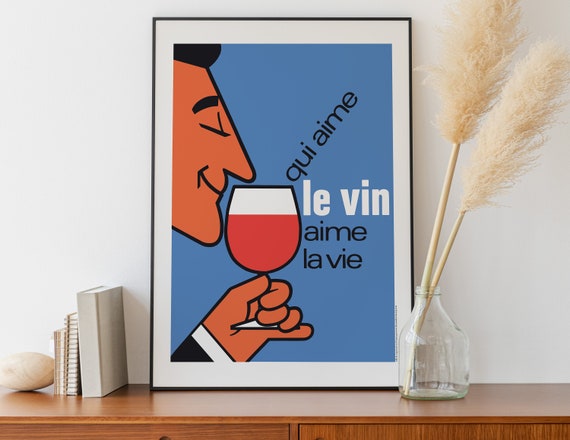This image depicts a photograph of a framed print sitting on a dark wooden shelf against a grayish-white wall. The main focus of the image is the colorful print featuring an animated man with brownish-orange skin, black hair, and closed eyes, smiling joyfully as he sniffs a glass of red wine with his left hand. The man is dressed in a black suit jacket and a white shirt, facing slightly to the right in profile.

The print includes a French phrase, "qui aime le vin, aime la vie," meaning "if you love wine, you love life." The words "le vin" are prominently displayed in larger white font, while the rest of the phrase is in black font.

The frame of the print is black with a white matte. The shelf also holds various objects: to the left of the print, there is a decorative rock acting as a bookend for three books, one of which is gray while the others have spiral bindings. To the right of the print, there is a clear vase with a couple of light brown, beige-feathered sticks arranged as decoration.